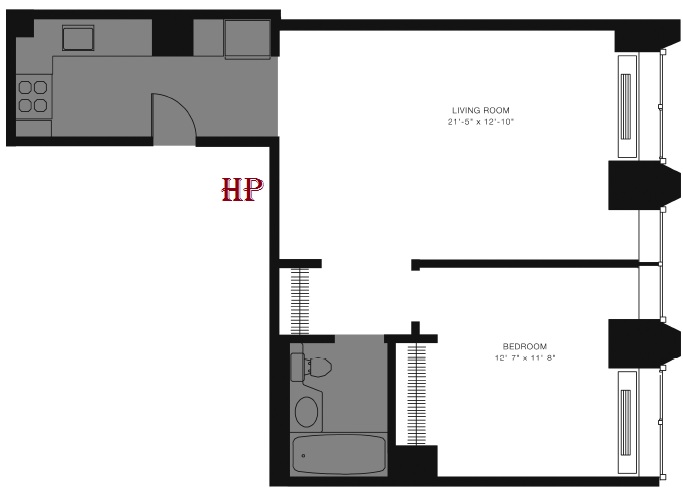This schematic illustrates the floor plan of a house, potentially depicting the loft area. Dominated by a spacious living room measuring 21 feet 5 inches by 12 feet 10 inches and a bedroom sized at 12 feet 7 inches by 11 feet 8 inches, both rooms feature windows that provide natural light and are situated above radiators. The bedroom includes a built-in closet, and an additional closet is accessible from the hallway adjacent to the living room. A shared bathroom, equipped with a bathtub, sink, and toilet, connects both the living room and the bedroom. On the left side of the schematic, there appears to be a kitchen area shaded in gray, suggesting it might be located on a lower level, though this is not explicitly confirmed by the illustration. Additionally, a red "HP" marking is visible on the plan, whose significance could range from a designer's initials to an annotation. The layout's detailed representation suggests versatility, hinting that it could be part of a hotel or similar lodging establishment.